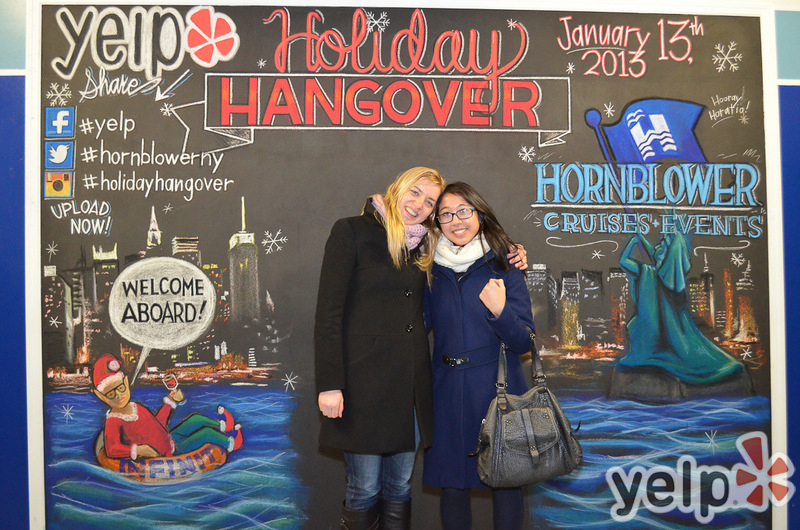This photograph features two women posing closely together in front of a vivid poster, with both of them leaning their heads together. The woman on the left sports blonde hair, a black jacket, blue jeans, and black boots. Next to her, the woman on the right has brown hair, black-framed glasses, and she is dressed in a purple coat with blue tights, accessorized with a large gray bag. 

Behind them, the colorful poster reads "Holiday Hangover" in striking red text at the very top. The left upper part of the poster has the Yelp logo, followed by a list of social media prompts: a Facebook icon with "#Yelp," a Twitter icon accompanied by "#HornblowerNY," and an Instagram icon with "#HolidayHangover." Below these, "Upload Now" is inscribed in black text. 

The poster also depicts a whimsical sand elf leaning in a donut floaty, cheerfully holding a wine glass and welcoming viewers with the text, "Welcome aboard," while some drawn skyscrapers are seen in the backdrop. On the right side of the poster, it states "January 13, 2013" and "Hornblower Cruises and Events" in smaller text. At the bottom right, the recognizable Yelp logo appears again, and in the distance, one can see the Statue of Liberty holding up a blue flag, adding to the overall holiday theme of the image.